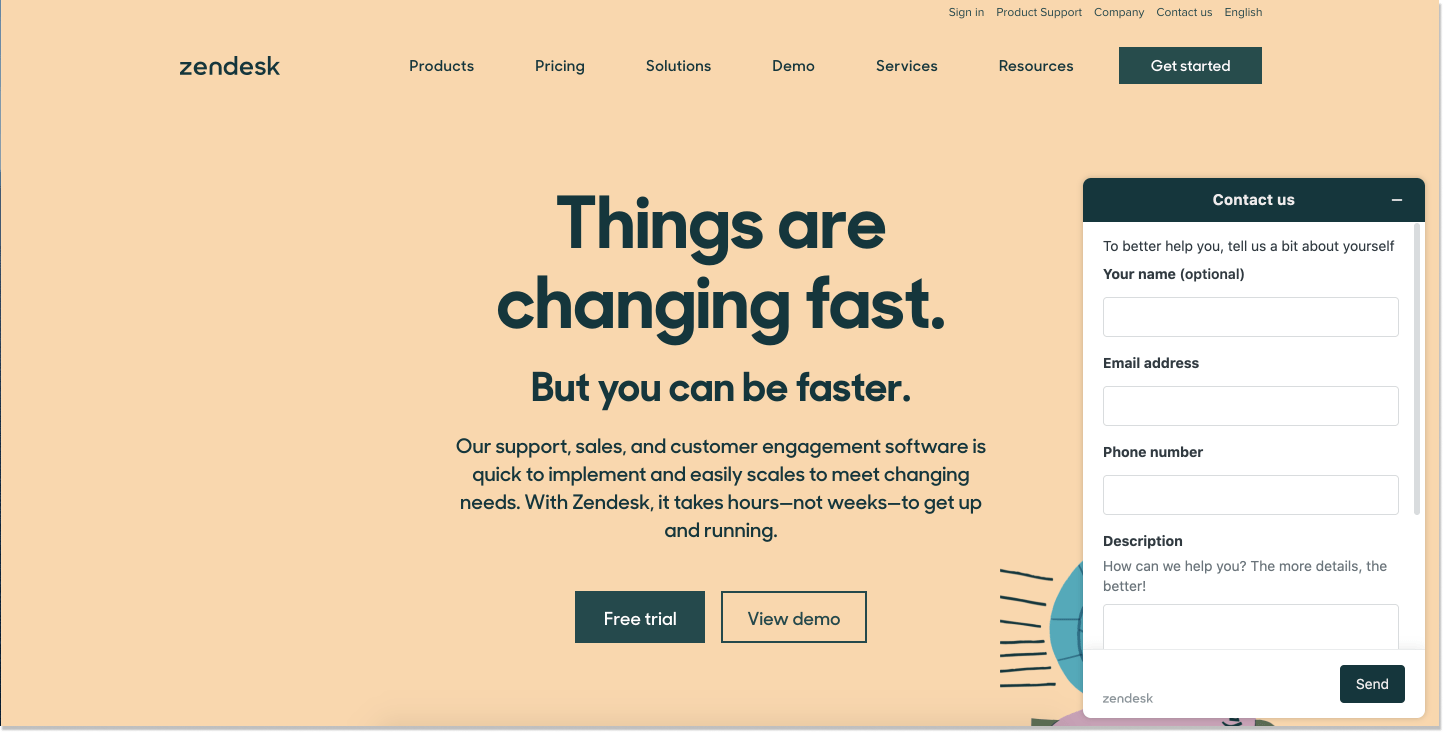The image showcases the login page of the Zendesk website, set against a brown background. At the top are several tabs labeled in English, including "Sign In," "Product Support," and "Company Contact Us." Beneath these, additional tabs are visible: "Products," "Pricing," "Solutions," "Demo Services," and "Resources."

Prominently displayed in the center is a black-text message that reads: "Things are changing fast, but you can be faster. Our support, sales, and customer engagement software is quick to implement and easily scalable to meet changing needs. With Zendesk, it takes hours, not weeks, to get up and running." Below this, there are two buttons, "Free Trial" and "View Demo." The "Free Trial" button is dark black, while the "View Demo" button is uncolored.

To the right, a contact form labeled "Contact Us" is positioned. The form begins with a prompt, "To better help you, tell us a bit about yourself," and includes fields for "Your Name (optional)," "Email Address," "Phone Number," and "Description." The description field asks, "How can we help you? Provide more details." At the bottom right of the form, a dark-colored "Send" button is available. On the bottom left of the form, the text "Zendesk" is displayed.